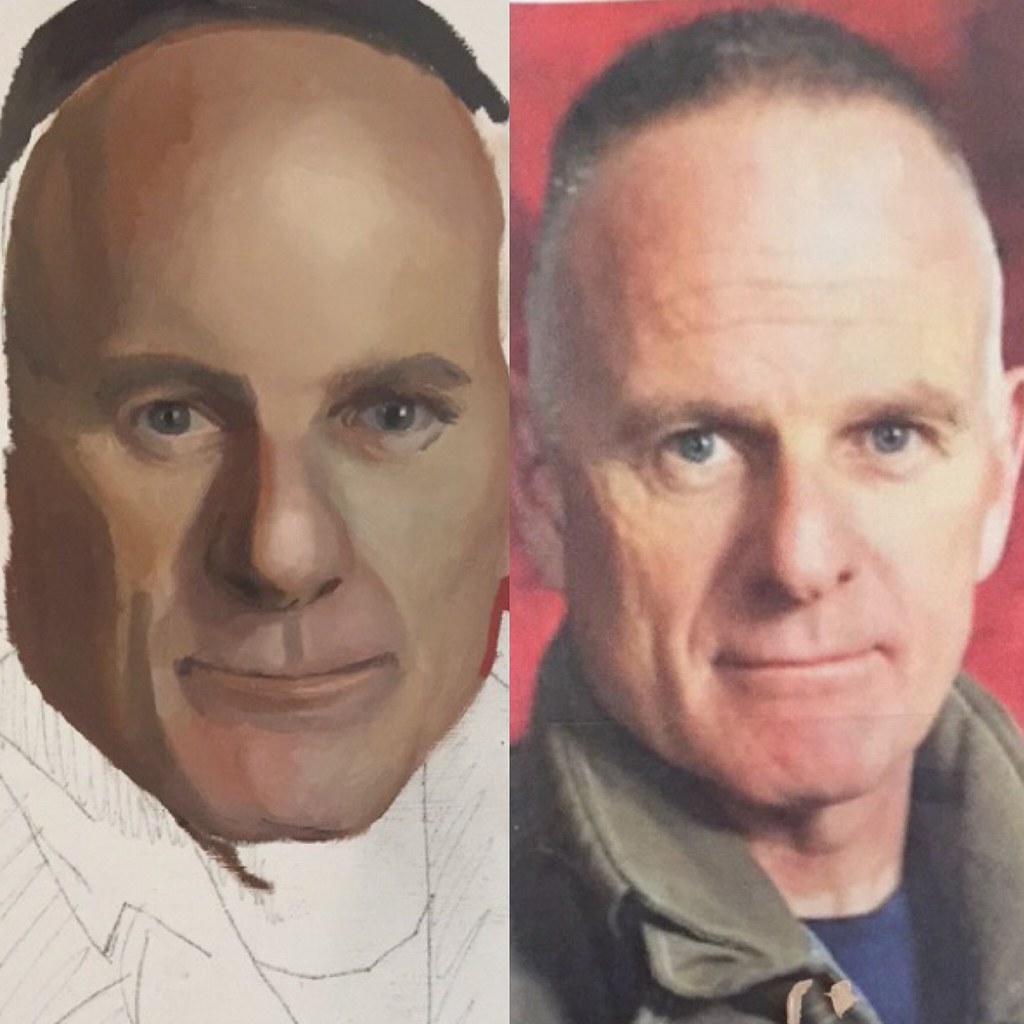The image depicts an artist's sketch in progress alongside the reference photograph of an older man, who appears to be in his late 50s or early 60s. The subject has a slightly balding head with dark hair on top and silver hair on the sides, complemented by blue eyes and bushy eyebrows. His face exhibits the natural creases and lines of aging. He is wearing a blue shirt and a green jacket.

On the left side of the image, the pencil drawing captures the beginnings of the man's likeness. The face is partially rendered, with perhaps the initial two or three layers of skin tone applied. The eyes are notably detailed and complete, though the hair seems to be floating above the head rather than anchored to it, indicating a work in progress. The outline of the jacket and shirt is present but remains in black and white, awaiting further detail and shading. Overall, the sketch shows promise and skill, vividly capturing the essence of the man's features while clearly being in the early stages of completion.